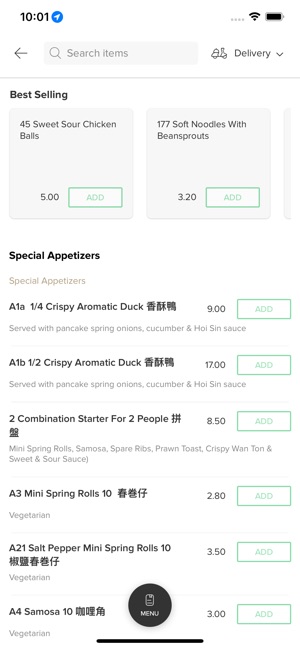The image is a close-up shot of a cell phone screen displaying a food delivery app, possibly showcasing Chinese cuisine. At the top, the phone's status bar is visible, showing a black print reading "10:01," a white airplane icon within a blue circle, and indicators for Wi-Fi connectivity and a fully charged battery, represented by a completely filled black battery icon. 

Below the status bar, there is a user interface element with a left-pointing arrow, a "Search items" field accompanied by a magnifying glass icon, a scooter icon labeled "Delivery," and several dots likely indicating a menu or pagination.

The main content of the screen features a section titled "Best-selling," which lists popular menu items with accompanying details. The first item is "45 Sweet and Sour Chicken Balls" priced at $5, with an "Add" button beside it. To the right, "177 Soft Noodles with Bean Sprouts" is listed for $3.20, also with an "Add" button.

Further down, under "Special Appetizers," the menu offers:
- A1: 1/4 Crispy Aromatic Duck for $9
- A1B: 1/2 Crispy Aromatic Duck for $17
- Combination Starter for Two People for $8.50

The menu continues with additional items, suggesting an extensive selection available for order.